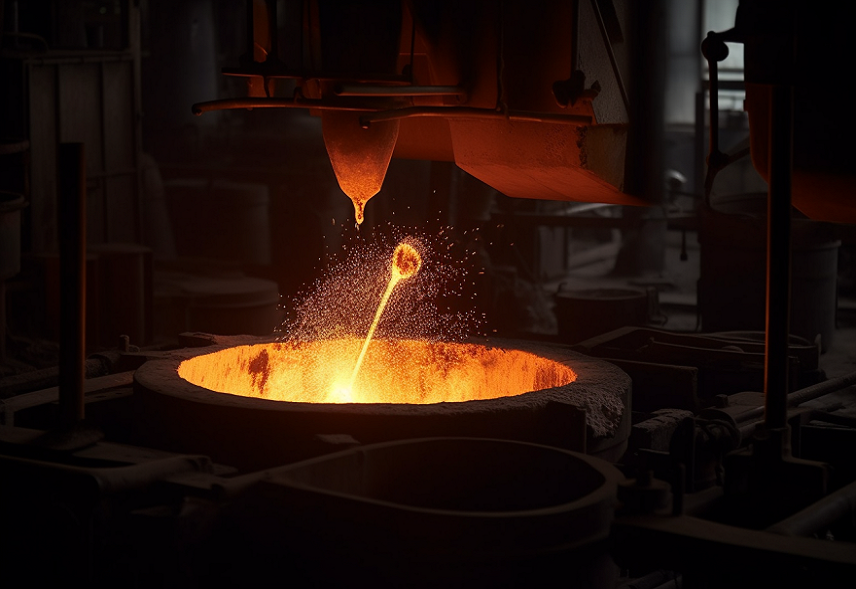The photograph captures an industrial, circular kiln or furnace, constructed from a rough but mostly smooth cement or brick material, designed to withstand extremely high temperatures. The scene is dim, with the primary light source emanating from the center of the kiln, where a molten hot liquid radiates a vivid reddish-orange glow. Rising above this liquid is a streak of bright yellow, culminating in a sphere of intense orange and yellow hues suspended in mid-air. Surrounding the kiln is an array of metal equipment, large pipes, bolts, and tools, whose details are obscured by the darkness. The image conveys the atmosphere of a melting factory, possibly for glass making or weapon forging, with no people present in the vicinity, emphasizing the intense heat and industrial nature of the environment.